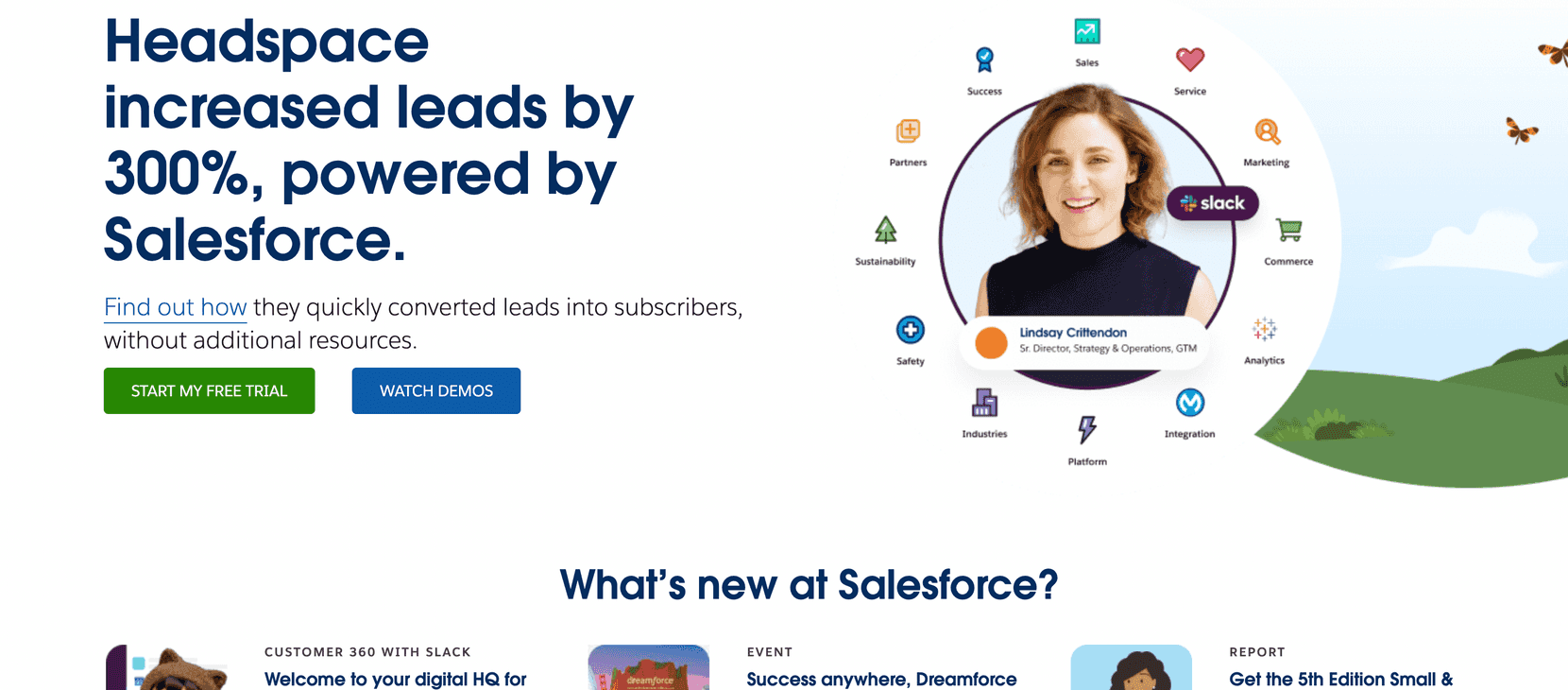This image is a promotional banner from Salesforce, emphasizing the significant success story of Headspace, which managed to increase its leads by an impressive 300%, thanks to the power of Salesforce. The banner invites viewers to "Find out how they quickly converted leads into subscribers without any additional resources," with a clickable hyperlink embedded in the text. Below this call to action, there are two prominent buttons: a green one labeled "Start My Free Trial" and a blue one labeled "Watch Demos."

To the right of the text, there's an image of a woman named Lindsay, engaged in a Slack conversation. Surrounding her are several icons representing various Salesforce offerings, including analytics, commerce, marketing, service, and sales. At the bottom of the banner, there's a partially cut-off message promoting various Salesforce features and events. It mentions "What's New at Salesforce," references "Customer 360 with Slack," and provides a glimpse of events and reports such as "Success Anywhere Dreamforce" and the "Fifth Edition Small and..." 

Overall, the banner serves as a detailed showcase of Salesforce's capabilities in driving substantial growth and productivity for its clients, paired with options to explore further through trials and demos.